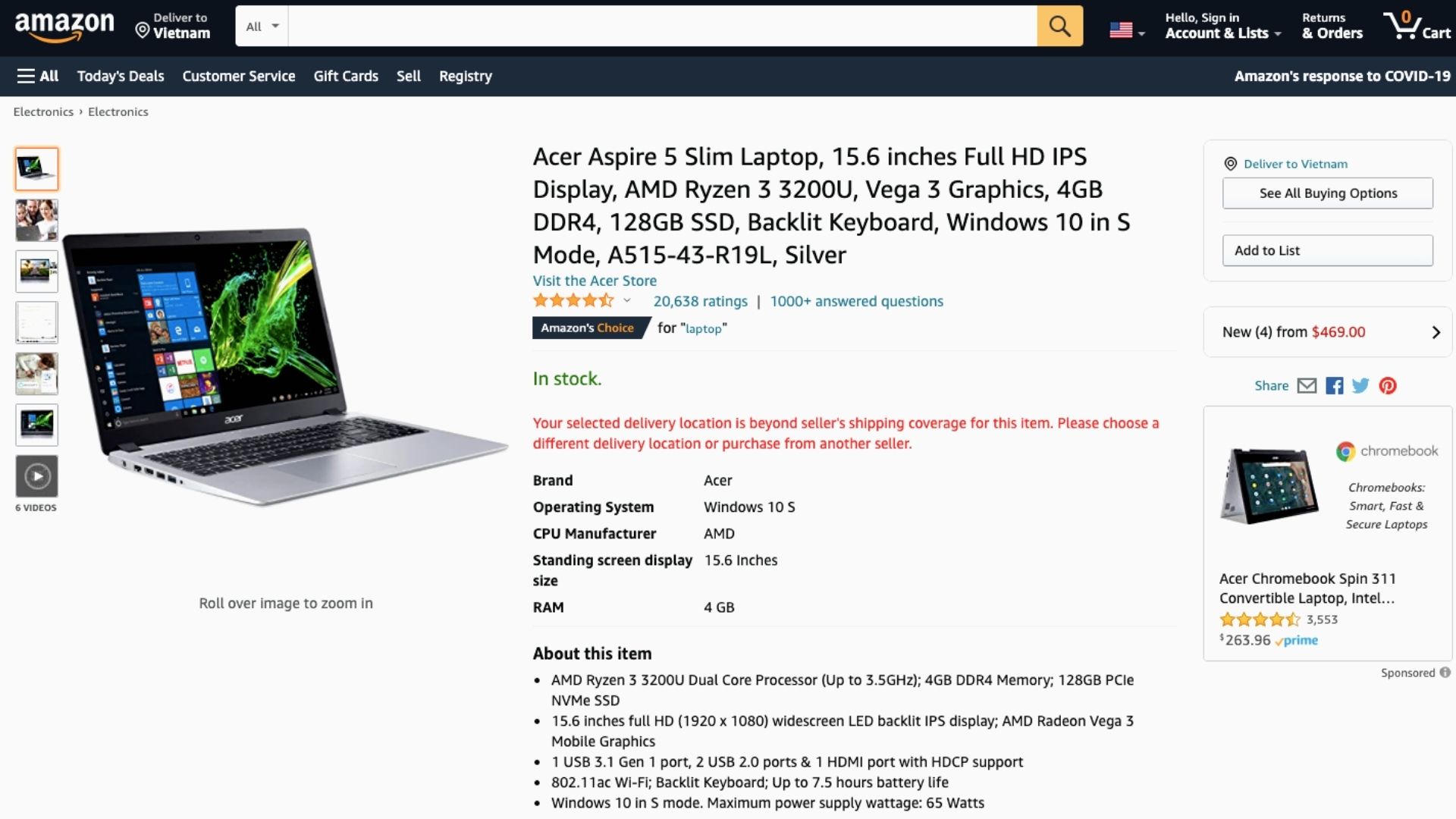The image depicts an Amazon.com webpage. At the top, the Amazon logo with its signature smiley arrow icon is prominently displayed. Next to it, the site confirms the delivery location as Vietnam. A search box with a drop-down arrow and the American flag symbolizing the English version of the site are visible. There is also a drop-down menu to change the country. To the right of these elements are various user account options including "Hello, Sign In Account & Lists" with a drop-down arrow, "Returns & Orders," and a shopping cart icon indicating zero items.

Below, a navigation bar includes tabs for "All" (indicated by a hamburger menu icon), "Today's Deals," "Customer Service," "Gift Cards," "Sell," and "Registry." The far right corner highlights Amazon's response to COVID-19.

The main section of the page features a prominent image of an Acer Aspire 5 Slim Laptop alongside seven smaller thumbnail images. This laptop boasts a 15.6-inch Full HD IPS display, powered by an AMD Ryzen 3 3200U processor with Vega 3 graphics, 4GB DDR4 RAM, and a 128GB SSD. It also features a backlit keyboard and runs on Windows 10 in S mode. The model number is A515-43-R19L in silver. The listing provides a link to visit the Acer store.

The product has garnered an impressive 4.5 out of 5 stars based on 20,000 ratings and is marked as Amazon’s Choice for laptops. However, it mentions that the selected delivery location in Vietnam is beyond the seller's shipping coverage. Users are advised to choose a different location or purchase from another seller.

Further down, product details are specified including the brand, operating system, CPU manufacturer, screen size, and RAM. Additional options include "See All Buying Options," "Add to List," and purchasing from "4 new from $469." Social sharing options are available for email, Facebook, Twitter, and Pinterest.